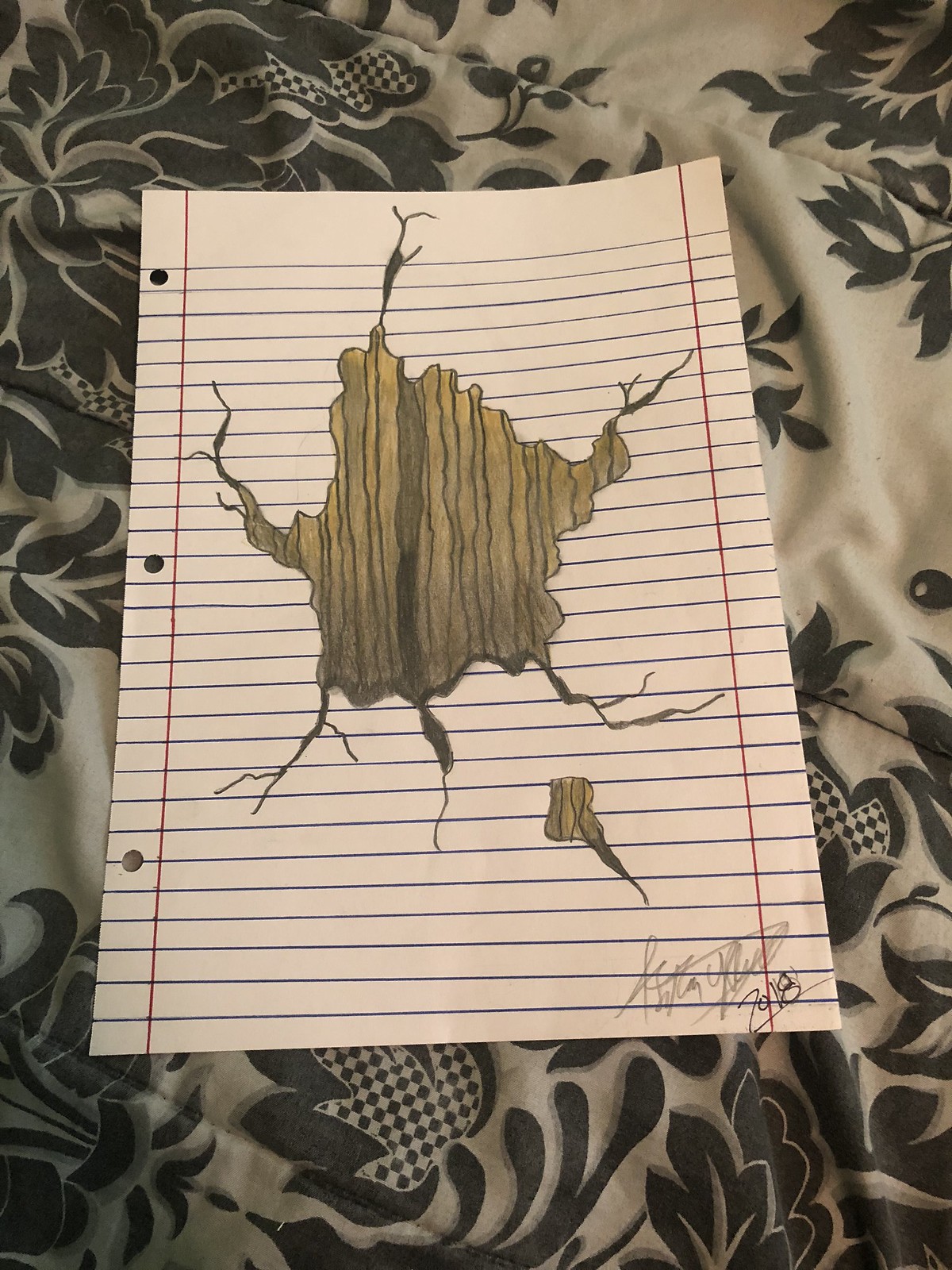A detailed image depicts a piece of lined notebook paper, complete with three-hole punches along the left side aligned vertically for binder placement. The paper features prominent blue horizontal lines and red vertical margins on each side. In the center of the paper is a drawing mimicking wood grain, which cleverly creates the illusion of a hole through which wooden texture is visible. This wood texture is composed of vertical lines in varying shades of brown, with the darkest shade in the middle and lighter tones towards the edges. Some parts of the drawing resemble roots extending outward. Below the drawing and to the right, a signature, including letters that look like a "U" and possibly an "H," is inscribed with the year "2018." All this is set against a backdrop of a soft, gray comforter adorned with a black leaf and floral pattern.